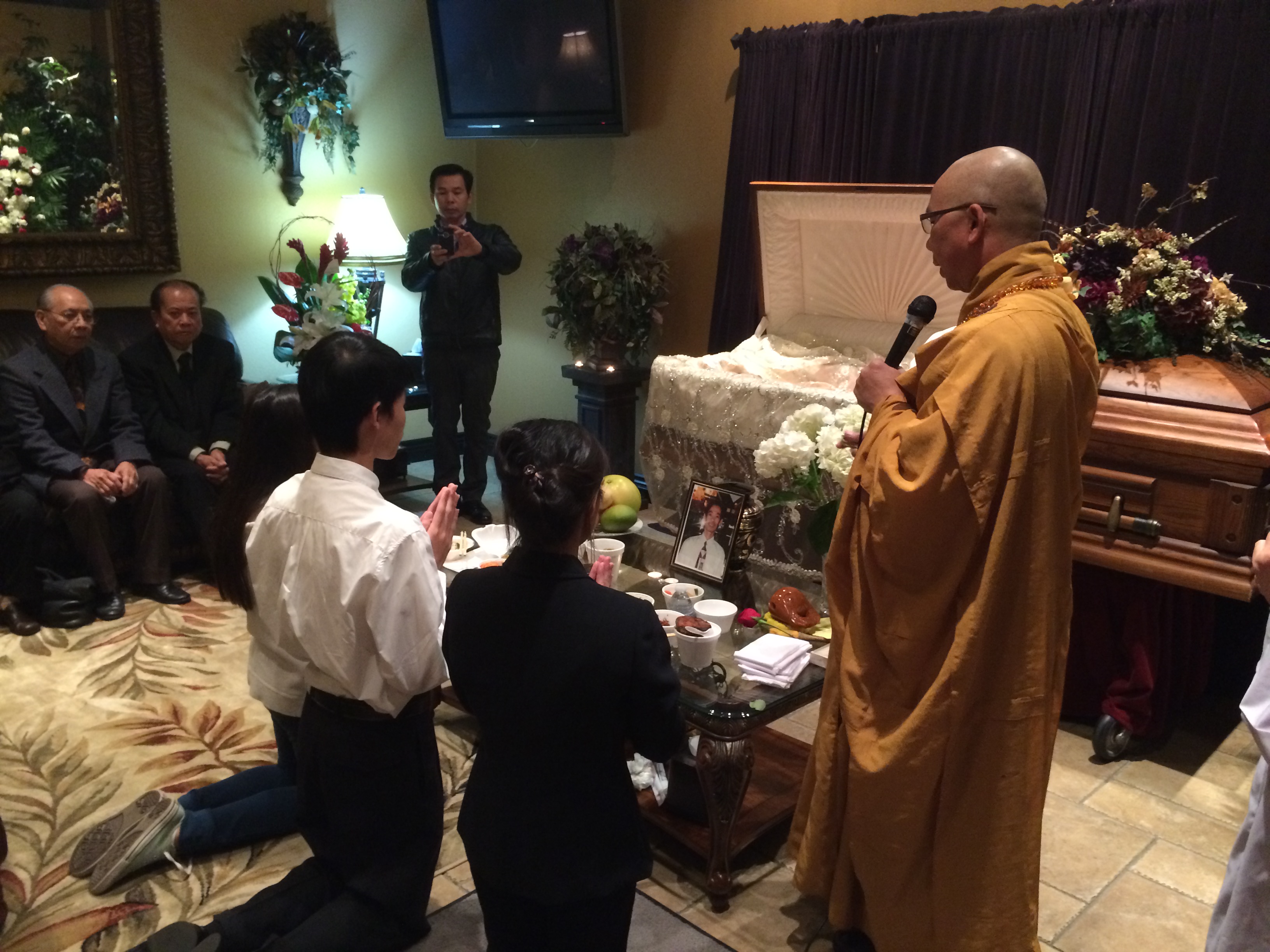This photograph captures a solemn funeral service. At the forefront, there is a medium brown wooden coffin, half-open and half-closed, covered partially with a white blanket, and adorned with a bouquet of flowers on the closed half. In the center, two people, likely part of an Asian family, are kneeling and praying in front of a table that holds a photo of the deceased man. To the right of them stands a bald priest or possibly a Buddhist monk, dressed in a light brown cloak and holding a microphone. Beside them, against the left wall, several people wearing suits are seated on a black leather couch, with a flower-patterned rug featuring beige, olive, and red hues under their feet. In the background, there is a person taking photographs of the kneeling individuals. The floor is tiled, and in the upper left-hand corner, a TV and a lamp are mounted on the wall. The room is also filled with multiple flower arrangements and vines, adding to the decor of the service.